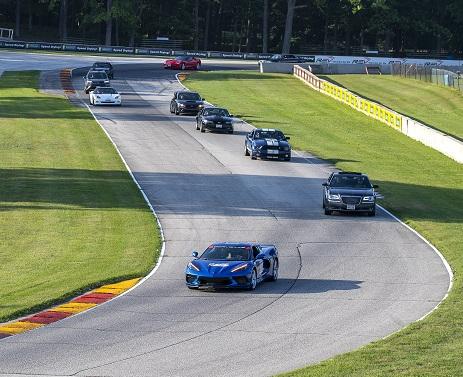This elevated photograph captures the excitement of a car race on a grey asphalt racetrack. The track starts from the bottom left-hand corner, curves to the left in the front, straightens out in the middle, and curves again towards the top right, creating a dynamic S-shape. The track is flanked by well-manicured green grass on both sides, and a fence is visible on the right.

Several cars are racing in two indistinct lanes, with a mix of blue, grey, white, and red vehicles. In the right lane, a blue sports car leads, followed by a white car, two indistinct ones, and a red car. The left lane features a dark blue car at the front and a black car trailing behind. Some of the cars, including the Mustangs, have distinctive design elements like slanted headlights with white strips.

In the background, the dense trunks of trees and glimpses of signs and banners provide a scenic backdrop, enhancing the outdoor racing atmosphere.